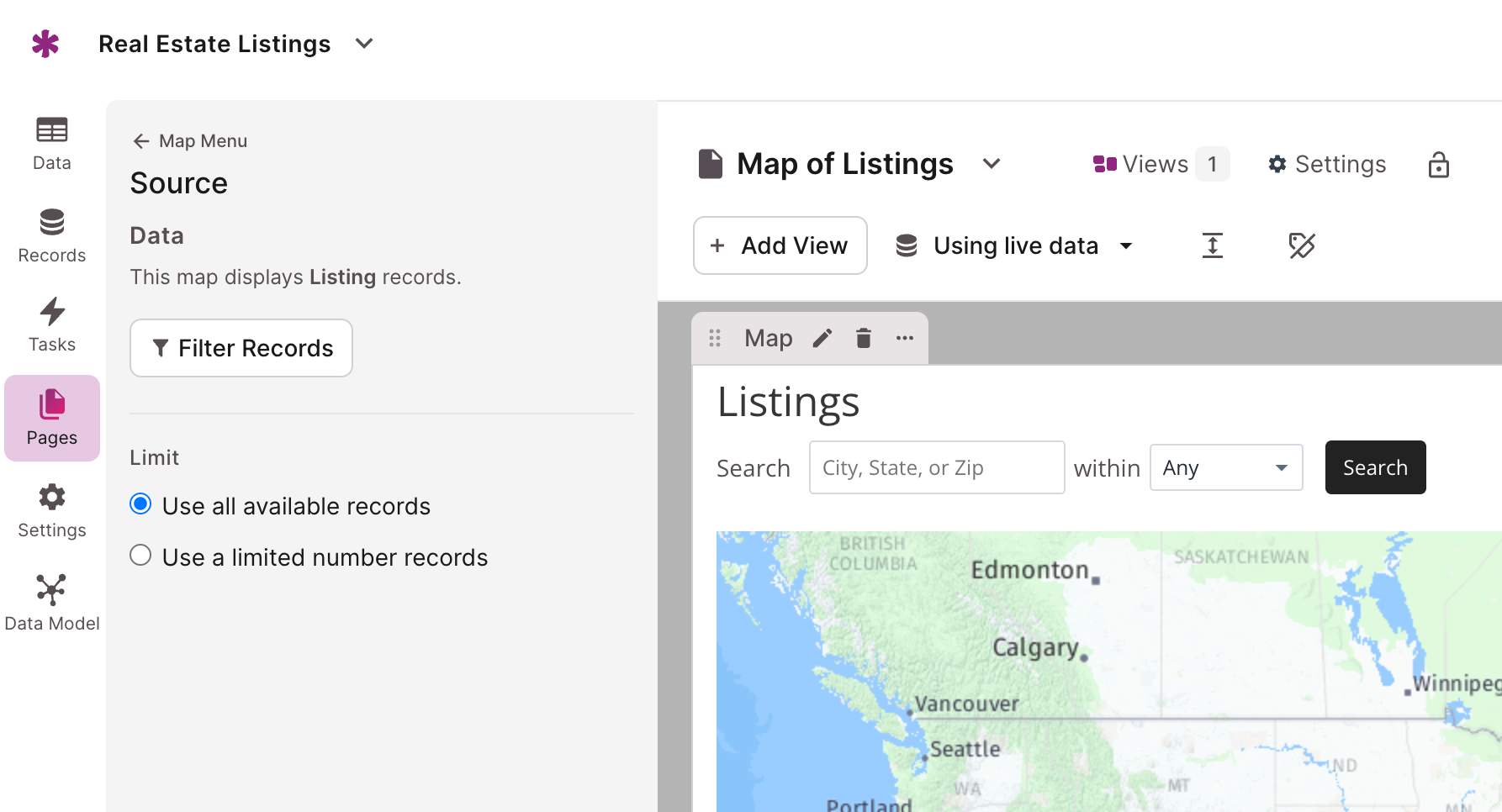This is a detailed caption for the screenshot:

---

The image captures a screenshot of a website or application interface primarily focused on real estate listings. In the upper left corner, there is a purple asterisk symbol. Next to it, prominently displayed, are the words "Real Estate Listings" with an accompanying drop-down menu. Running vertically down the left side of the screen is a navigation menu with the following options: "Data," "Records," "Tasks," and "Pages" (which is currently highlighted), followed by "Settings," and "Data Model." 

To the right of this vertical menu, there is a back button represented by an arrow icon, and next to it, the text "Map Menu." Below that, you'll find the word "Source," followed by the label "Data." An explanatory text reads, "This map displays listing records." Further down, there is a "Filter Records" button next to a limit option that presents two choices: "Use all available records" (which is selected) and "Use a limited number of records" (which is not selected). 

To the right of this section, there is a heading that reads "Map of Listings" along with a drop-down arrow. Below it are indicators for "Views 1," a settings button, and an "Add View" button that includes a drop-down menu for "Using Live Data." 

In the main content area of the screen, there is a map focused on the Pacific Northwest, specifically showcasing regions around Vancouver, Canada, and Seattle, Washington.

---